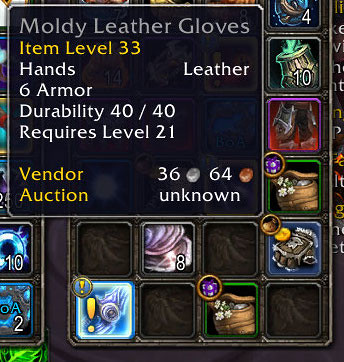This is an up-close screenshot of a mobile phone game, showcasing item details and inventory icons. The focal point is a black rectangle outlined in white, containing detailed information about "Moldy Leather Gloves". "Moldy Leather Gloves" is prominently displayed in light gray text, followed by "Item Level 33" in yellow. Below, it states "Hands, Leather" in white and "6 Armor" indicating the item's defense value. The gloves have "Durability 40/40" and "Requires Level 21" to equip. At the bottom left, "Vendor" is highlighted in yellow, with "36 silver, 64 copper" depicted as small circle icons, and "Auction Unknown" is mentioned in white.

On the right side of the image, there are several small squares with various images and numbers, indicative of different game items. These include a pair of brown gloves over a blue background with white accents in a dark gray square, a light brown leather satchel with white flowers in a green square, a pair of pants in a purple square, and a vase with green liquid in a silver square. Additionally, there are small tiles showing numbers like "4" and "10" with colorful jewels, namely a purple and yellow jewel. At the bottom center, there is a blue square with a prominent yellow exclamation point, and nearby, a circular icon with a similar exclamation point. There are also blue-tinted images with numbers "10" and possibly "2" near the bottom left corner.